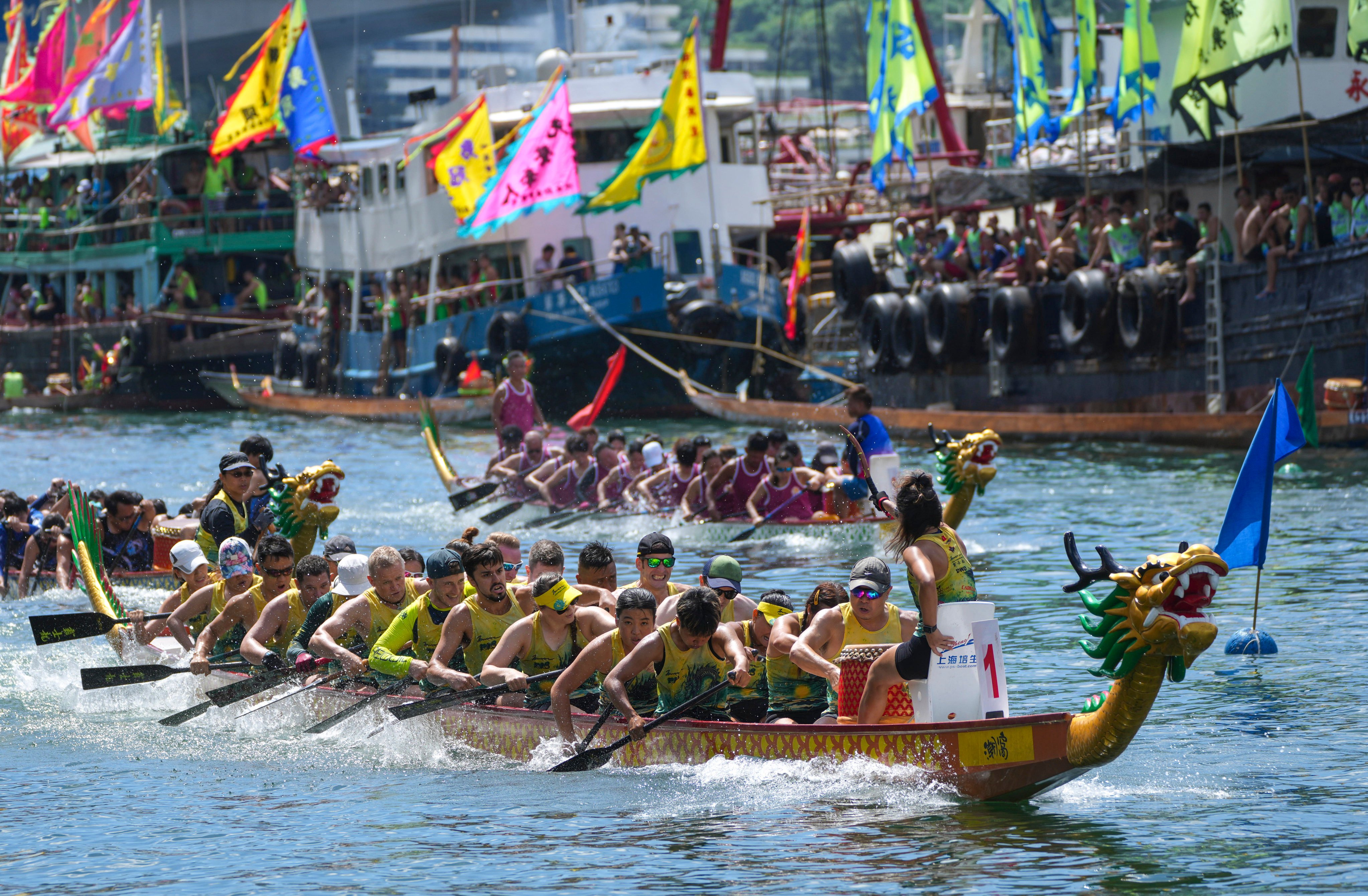The image captures a vibrant dragon boat race set in an Asian harbor, characterized by multiple sleek, canoe-like boats each adorned with intricately designed dragon heads. These dragon heads are primarily yellow with green accents. The scene showcases three teams fiercely competing: a leading yellow team, a purple team, and a third team in various colors, possibly blue. Each team consists of several rowers in matching uniforms, followed by a coach or drummer in the front. The yellow team, with around eleven members, rows with black oars and is currently ahead, passing a significant blue floating marker which might signify a checkpoint or victory.

In the foreground, the yellow team's boat is the most prominent, pointing right with the dragon’s head clearly visible. The rowers are coordinated in yellow tank tops and black shorts. The purple team can also be seen, though slightly further back. Alongside the race, numerous larger ships are moored, carrying enthusiastic spectators. The closest ship is black with black tires used as bumpers, while others feature varying color schemes including blue, white, and green. These spectator ships are festooned with a multitude of flags in green, yellow, and pink, adding to the festive and competitive atmosphere of this vibrant cultural event.